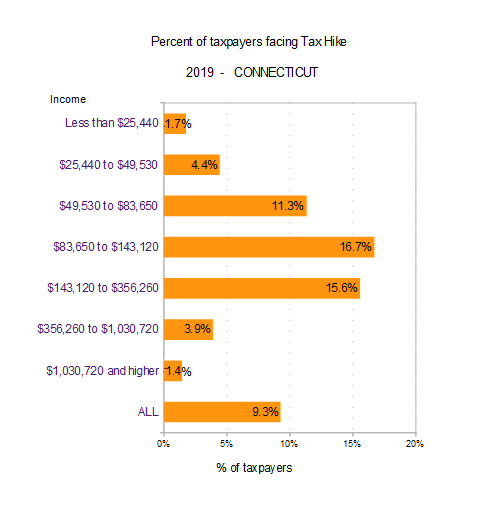The image is a line chart titled "Percent of Taxpayers Facing Tax Hike in 2019-19 Connecticut." The y-axis represents the percentage of taxpayers, ranging from 0% to 20% in 5% increments. The x-axis represents different income levels, starting from "less than $25,440" at the top and ending with "All" at the bottom. The chart features an orange line indicating the percent of taxpayers facing a tax hike at various income levels: less than $25,440 is 1.7%, $25,440 to $49,530 is 4.4%, $49,530 to $83,650 is 11.3%, $83,650 to $143,120 is 16.7%, $143,120 to $356,260 is 15.6%, $356,260 to $1,037,020 is 3.9%, $1,037,020 and higher is 1.4%, and for "All" income levels, it is 9.3%.